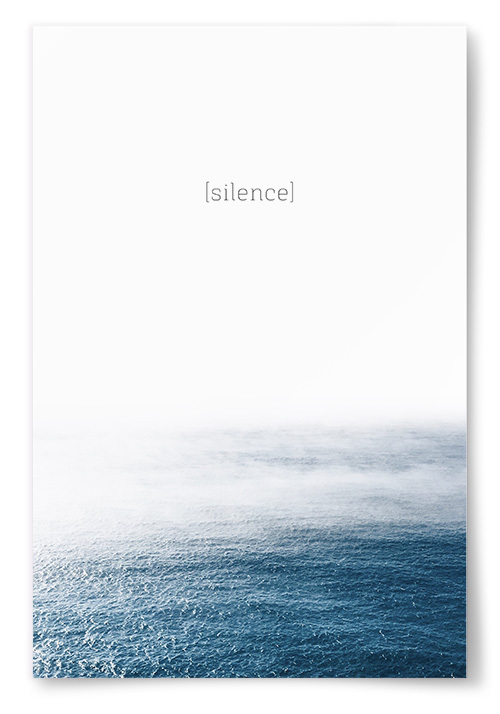The image is a vertical piece of artwork that conveys a sense of calm and meditation. The composition is divided into two distinct sections. The bottom third of the image features a tranquil, dark blue ocean that transitions into a teal shade, with a layer of mist gently hovering over the water. This portion of the image fades into a subtle gray tone on the horizon. The top two-thirds of the image is completely white, creating a stark, serene backdrop. Near the upper section, centrally placed within the white area, is the word "silence" in lowercase gray font, enclosed in brackets. The clean, minimalist design, combined with the ocean's stillness and the mist, evokes a profound sense of quiet and reflection. No additional objects or text are present, emphasizing the intended peaceful atmosphere.